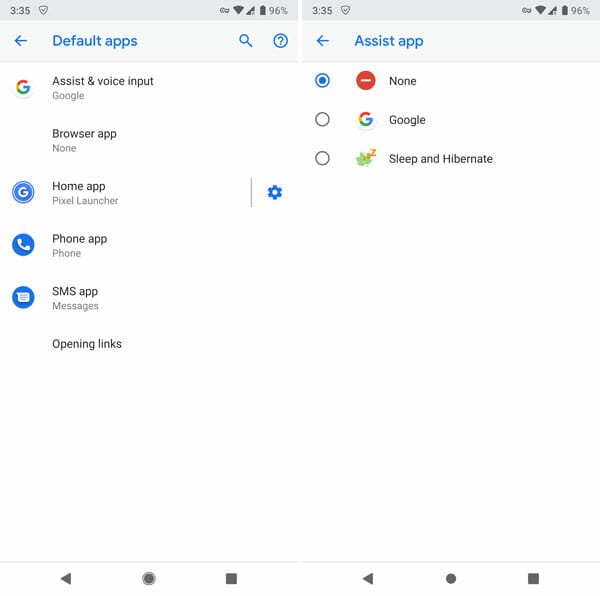The image displays two side-by-side mobile phone screen screenshots. Both screenshots show the same status bar at the top, which features the current time "3:35," a protective shield icon, a key icon, Wi-Fi and signal strength indicators, battery power, and battery percentage at "96%." Below the status bar, each screenshot has a gray box with blue text and a blue arrow pointing to the left. The first screenshot is titled "Default Apps," featuring a search icon and a question mark in blue. The second screenshot is marked "Assist App," also with a left arrow.

In the first screenshot, a list of default apps is presented, which includes:
- "Assist & voice input" with the Google icon
- "Browser app" listed as "None"
- "Home app" showing the blue and white G with the Pixel Launcher text
- "Phone app" with a white phone icon in a blue circle
- "SMS app" denoted as "Messages" with a message icon in a blue circle
Additionally, there is a section titled "Opening links."

The second screenshot focuses on selecting the default assist app, displaying a radio button menu:
- "None" marked by a selected radio button with a red circle and a white dash
- "Google" next to the Google logo, unselected
- "Sleep and hibernate" with its respective icon, also unselected